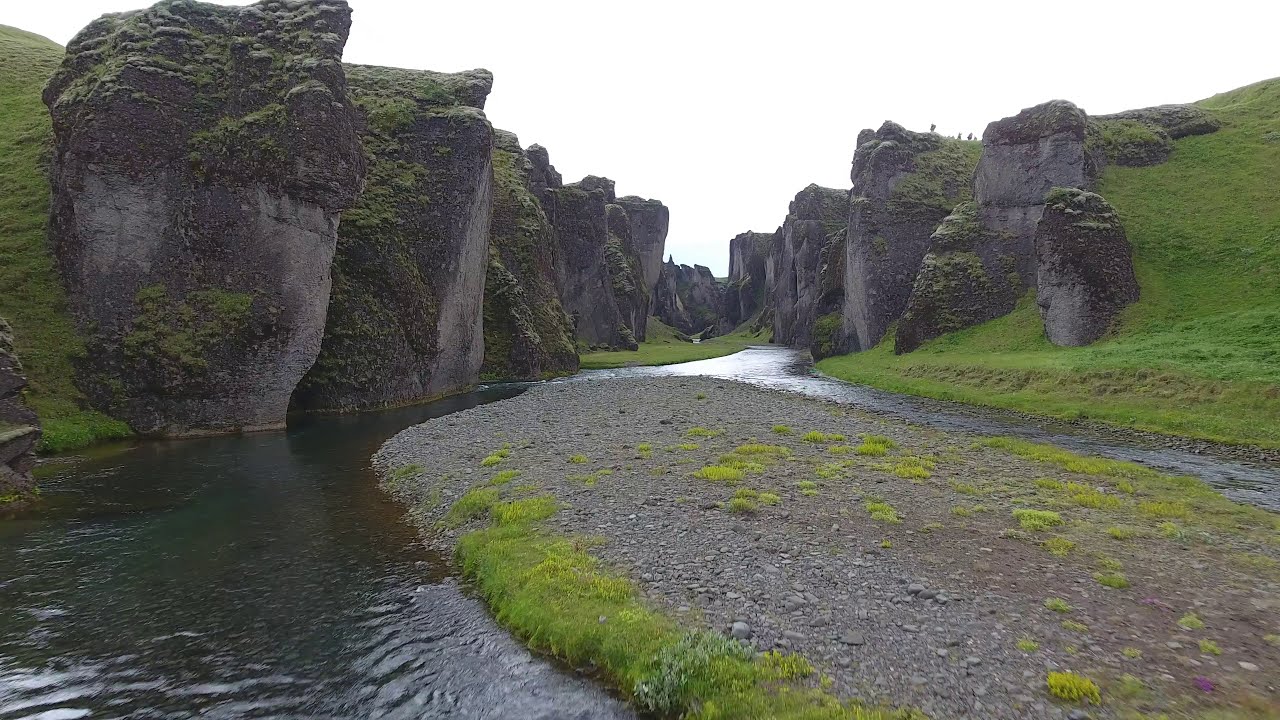This photograph showcases a stunning natural rock cavern made of dark gray granite, with a waterway winding through its midst. The sky above appears clouded and foggy, casting a stark white backdrop that enhances the sharp relief of the tall, angular rocks. The rocks on the left side of the image are particularly prominent, forming a dramatic foreground, while the rocks on the right gradually diminish in size, positioned on a grassy hill that slopes upward to the upper right edge of the frame.

From the center of the horizon, the river splits and winds through the cavern, creating an island in the middle about 20 yards long, covered in gravel and dotted with patches of green grass and vegetation. This island can be accessed from the bifurcation of the waterway, which extends from the center of the photo towards the foreground and left side. The cavern's rocky formations resemble cliff heads, standing approximately 50 feet tall and numbering around ten in the image, contributing to a valley-like setting.

Lush green vegetation grows out from various crevices in the rocks, adding color and life to the rugged landscape. This scene, reminiscent of terrains found in countries like Iceland or Switzerland, evokes a sense of serene, untouched nature, with the cold water winding its way around the ancient stone structures.